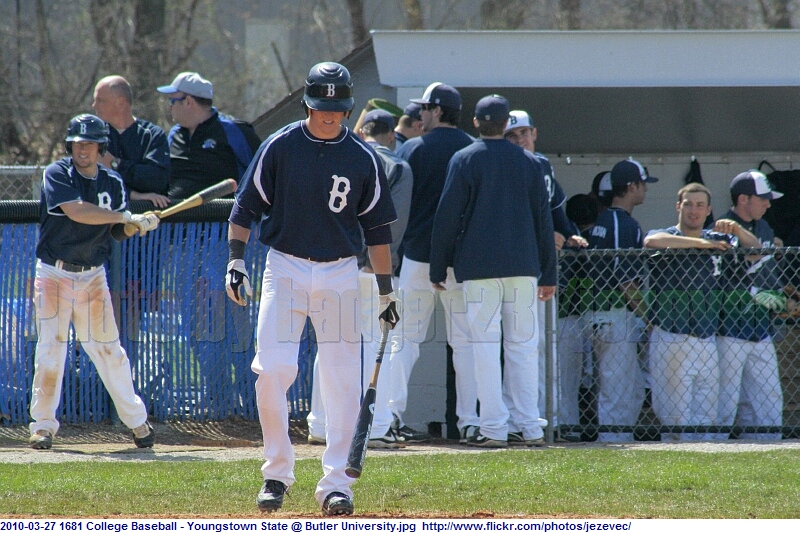The image depicts a scene from a college baseball game featuring players from Youngstown State and Butler University dated 2010-03-27, as indicated on a white border with blue writing below the picture. In the forefront stands a man wearing blue shirts and white pants, holding a bat angled down by his leg. Both he and another man on the field, who holds a bat in a swinging motion, are equipped with black helmets marked by white letter 'B's. The players also wear cleats, and there is visible dirt on the pants of the swinging player. A fence runs behind these men, segmenting the field from the dugout area where additional team members congregate. Behind the fence, approximately seven men can be seen, some interacting with players on the field, while others look on or rest their arms on the fence. The entire scene is set on a grassy baseball field.